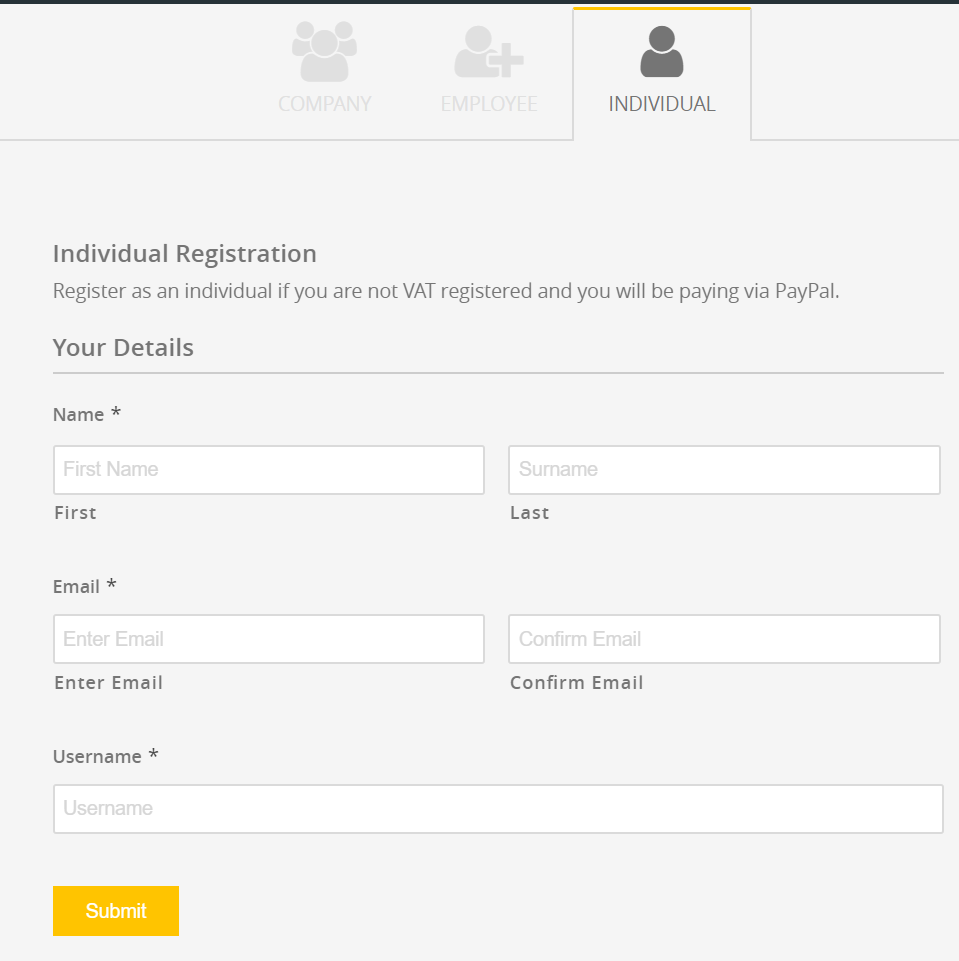The image depicts a screenshot of a registration page featuring three tabs at the top: "Company," "Employee," and "Individual." The tabs are represented by icons: the "Company" tab depicts three human silhouettes, the "Employee" tab shows a human silhouette with a plus sign, and the "Individual" tab displays a single human silhouette. The "Individual" tab is currently open and highlighted in dark gray.

The page is titled "Individual Registration" and includes a note stating that the registration is intended for individuals who are not VAT registered and will be paying via PayPal. The form within this page contains several fields labeled "Your Details," requiring information such as First Name, Last Name, and Email (entered twice for confirmation). There is also a field for creating a Username. Each required field is marked with an asterisk.

At the bottom left corner of the form, there's an orange "Submit" button with white text. The background color of the section is light gray, providing a clean and neutral backdrop. Additionally, the chart's top border features a bold black horizontal line, while subsequent lines are less prominent.